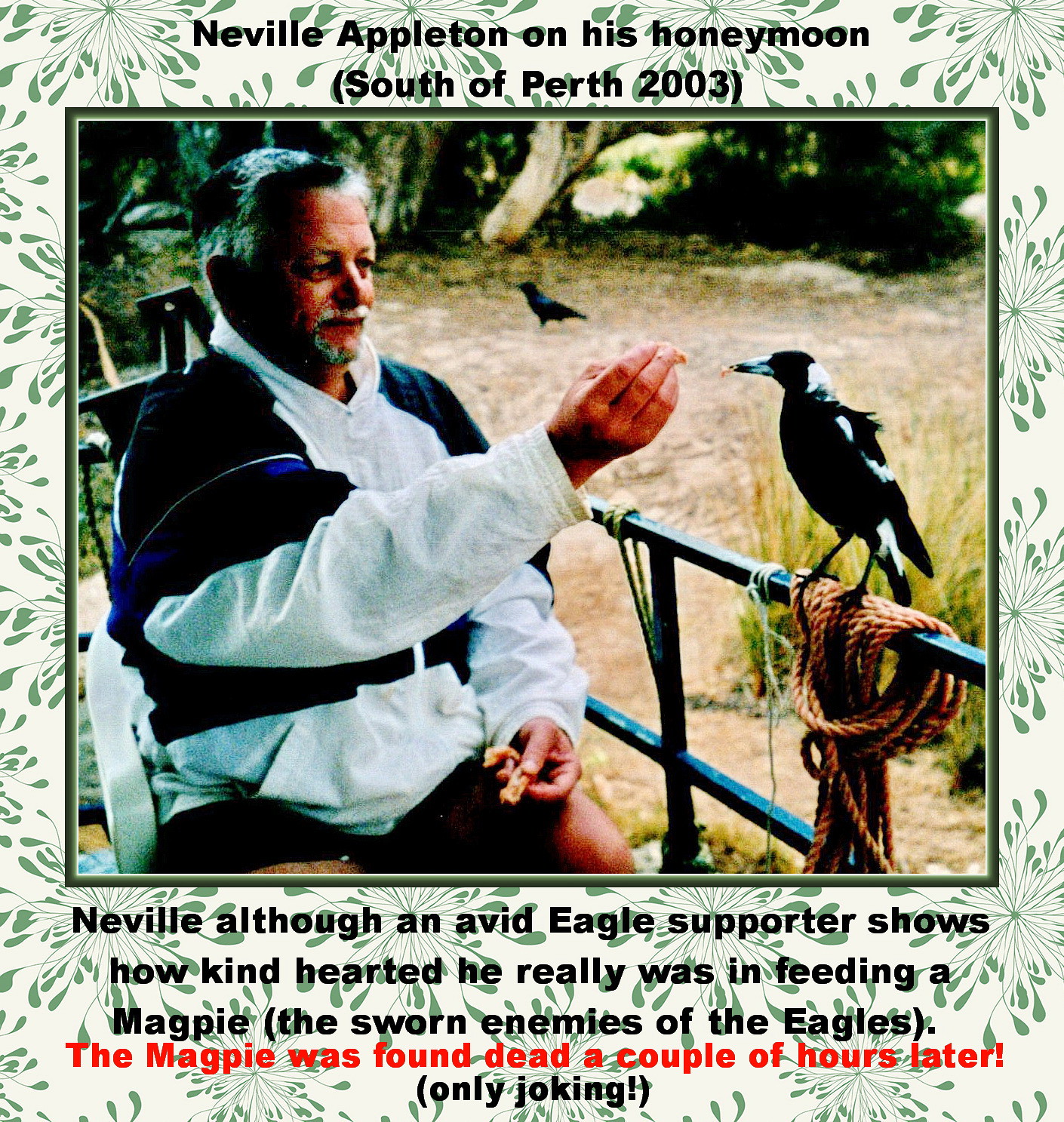This color photograph, surrounded by a cream background with green foliage, prominently features an older man identified by the black text above the image as "Neville Appleton on his honeymoon, South of Perth, 2003." Neville, seated and dressed in a light heather gray and black sweater with shorts, has grayish-white hair. His left arm is extended to feed a magpie, a black bird with white markings on its neck, back, and tail feathers, which is perched on a railing beside him. Intriguingly, a second all-black bird can be seen walking in the background amidst some trees and dirt ground. The railing features roped components reminiscent of a boat setting. Beneath the photo, an additional caption humorously notes, "Neville, although an avid Eagle supporter, shows how kind-hearted he really is in feeding a magpie, the sworn enemies of the Eagles," followed by a red text jesting, "the magpie was found dead a couple hours later," and finishing in black with "only joking."